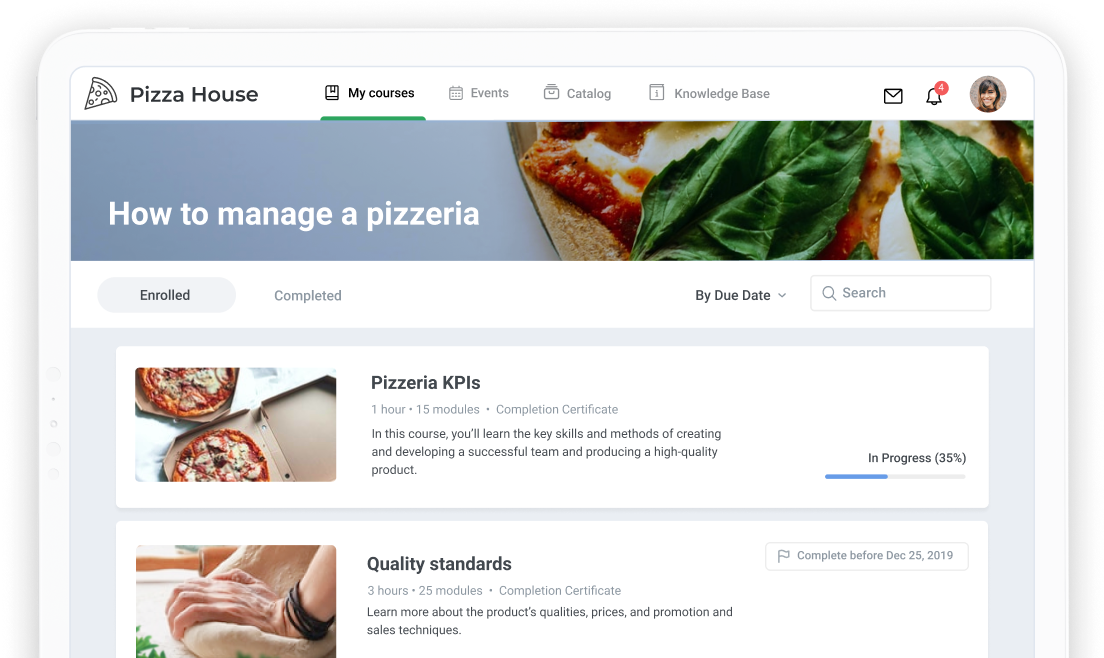A tablet display showcasing the "Pizza House" online learning platform. The tablet features a white rounded bezel, housing the website interface. In the top left corner, a pencil or pen-drawn slice of pizza sits next to the brand name "Pizza House." Adjacent to this logo, there's a navigation menu listing: My Courses, Events, Catalog, and Knowledge Base.

On the upper right, the interface displays a mail icon, an alert icon, and a user avatar. Below the navigation bar, a prominent banner with a gray background and several pictures of pizzas reads "How to Manage a Pizzeria."

Directly under the banner, the interface includes filters and search options: Enrolled, Completed, By Due Date, and Search, with "Enrolled" currently selected (highlighted in gray). 

The main content area shows two visible courses. The first course, "Pizzeria KPIs," is listed with details: 1 hour duration, 15 modules, and offers a Completion Certificate. The course description reads, "In this course, you’ll learn the key skills and methods of creating and developing a successful team and producing a high-quality product." To its right, there's a progress bar indicating 35% completion with a blue bar and text reading "In Progress."

Below this, the second course titled "Quality Standards" has a duration of 3 hours, 25 modules, and also includes a Completion Certificate. The accompanying description states, "Learn more about the product qualities, prices, and promotion sales techniques." This course has a deadline noted as "Completed before December 25th, 2019."